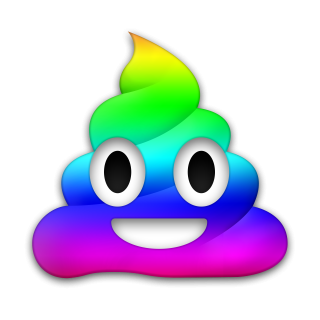The image features a popular emoji known as the poop emoji, presented in a vibrant rainbow gradient. Set against a plain white background, the emoji starts with a vivid bright pink at the base, transitioning smoothly through royal blue, light green, bright neon green, yellow, and finally to an orange crown at the tip. The emoji maintains its classic features with large, expressive white eyes with black pupils, and a cheerful smile. This computer-generated image, resembling a whimsical swirl akin to a snow cone or ice cream, creatively reimagines the poop emoji in a spectrum of colors, making it both playful and visually striking.